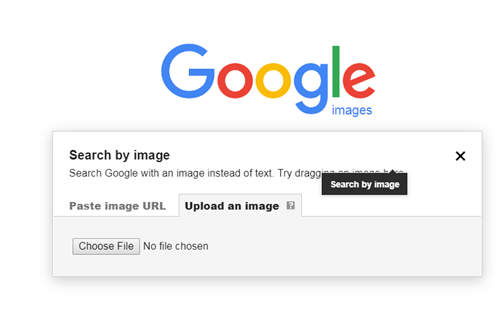The image is a screenshot of the Google Images website interface. At the top, the Google logo is prominently displayed, with "Google" rendered in its usual blue, red, yellow, and green colors. The word "Images" appears in dark blue next to the logo. 

Below the logo, there is a rectangular box with black text at the top saying "Search by image." This text is followed by the instruction, "Search Google with an image instead of text." An 'X' icon is to the right, which users can click to close this box. 

Further down, the interface provides two main options for image searching: "Paste image URL" and "Upload an image." Under "Upload an image," there is a button labeled "Choose file" to allow users to upload an image from their device, though currently, it indicates "No file chosen."

Above the "Upload an image" section, there is a black rectangle with white text that says "Search by image," partially obscuring some of the underlying text in the screenshot.